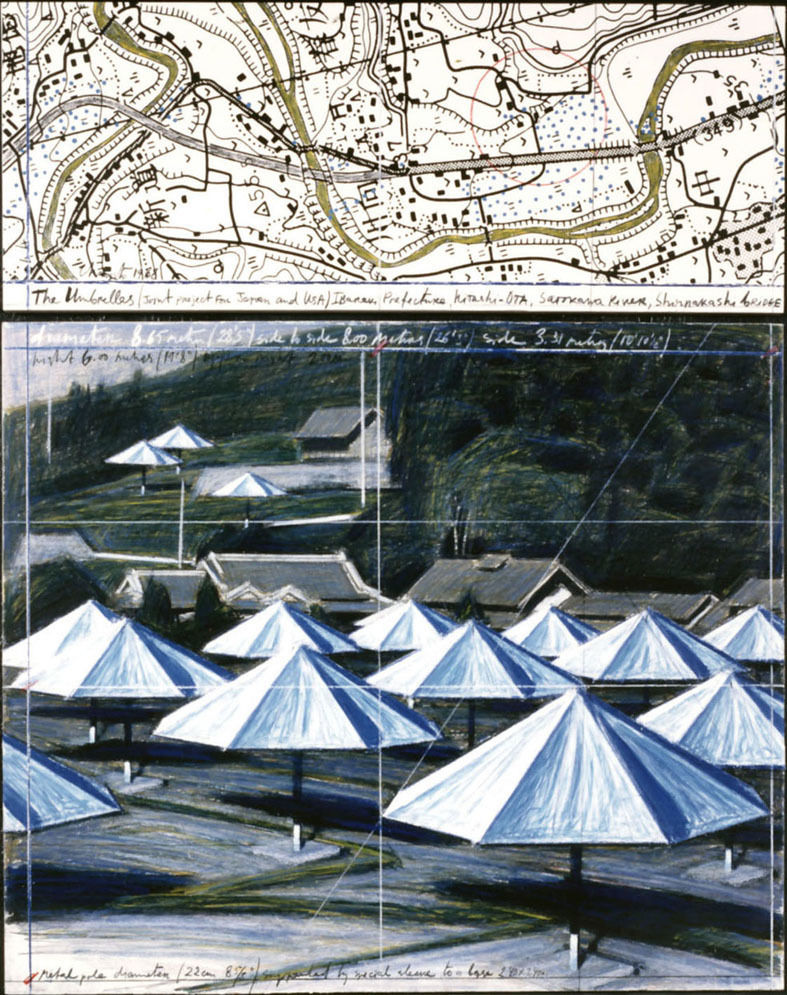This detailed painting is a color illustration combining elements of an old map and an architectural sketch. The top portion of the canvas features a rectangular, topographical map adorned with brown, squiggly lines that intersect at various angles, possibly representing roads or rivers. The map showcases numerous dots, curves, and circles indicative of city planning, and contains both non-English writing and numbers like 3, 4, and 9, though the script is too faint to interpret. Below the map is handwritten text that adds to the antique feel.

The bottom portion, occupying two-thirds of the image, vividly depicts a field filled with twelve partially-opened, white umbrellas standing upright on square bases, casting slight blue shadows. These umbrellas are set against a backdrop of gray-roofed houses and a lush green hillside. The hillside features additional umbrellas, detailed foliage, and more homes peeking through the dense trees. The detailed renderings of the leaves, shadows, and architectural elements highlight the interplay of man-made structures within a picturesque, natural landscape. Hatch lines throughout the illustration suggest dimensions and form, blending the intricate details of the setting with the map above.